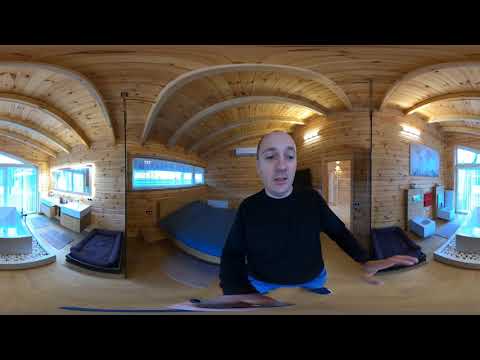This is a detailed 360-degree panoramic image showcasing a room with interconnected bathroom and bedroom areas. The room is distinctly characterized by its extensive wood paneling, rounded ceilings, and generally light yellow hue. Dominating the scene is a man of Caucasian descent, bald except for some brown hair on the sides, wearing a long-sleeved black shirt, blue jeans, and black shoes. He stands in the center of the room with his left hand raised as if signaling "stop."

To the left of the image is the bathroom, designed with both stone features and pebbled accents encircled by a small wall. The bathroom area includes a bathtub adjacent to a large window, allowing ample natural light. Parallel to the bathtub, there are two sinks with lighted mirrors above them. 

The background features a bed with a blue bedspread and a large glass door that offers an outside view. Directly behind the man, a window sits to the left of the bed, allowing additional light, and to the right, an open door leads to another part of the house, revealing a shower stall. The image stitching causes an optical illusion, making the walls appear bubbled outward and the top seams beveled, while the proportions at the lower part create a stretched appearance on objects like the man's hands and legs.

On the far left of the bathroom area, a picture hangs on the wall, and beneath it, there's possibly a pet bed. The wooden crossbeams above and area rugs on the floor contribute to the warm, rustic ambiance of the room.